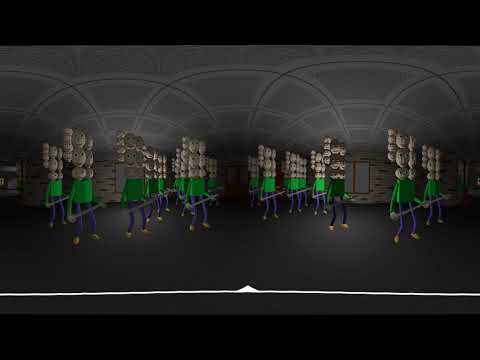In this digitally created image, we observe a peculiar indoor setting featuring an array of bizarre, computer-generated figurine characters. The image is framed by a black border, emphasizing the central scene. The environment is minimalistic, with a dark gray floor, and gray walls and ceiling, giving it an enclosed, somewhat stark atmosphere.

At the center, positioned deliberately, stand multiple humanoid figures that blend characteristics of stick figures and Lego characters. Each figure is composed of a slightly trapezoidal green torso and long, stick-like arms and legs in blue. Uniquely, these figures do not follow conventional human anatomy; instead of a single head, their torsos support an intricate arrangement of heads—two heads side-by-side, with additional heads stacked vertically above, summing up to six or seven heads per figure. The expressions on these heads vary from happiness to sadness to surprise.

Each character holds a wooden stick or bar, and their postures suggest a dynamic motion, almost as if they are mid-dance amidst the otherwise empty room. The distinct yet repetitive styling evokes the impression of a budget video game or a stylized animated scene. The palette consists primarily of black, gray, light gray, green, blue, and white, contributing to the overall surreal and slightly whimsical visual narrative.